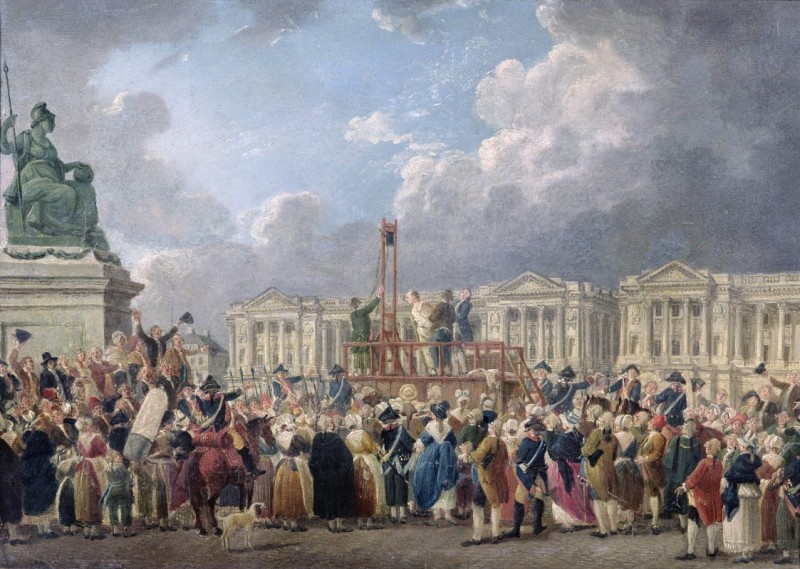In this watercolor-style painting reminiscent of Renaissance art, a dramatic execution scene unfolds under an overcast sky with dark, foreboding clouds. At the center, a bald man dressed in white stands on a raised platform, held firmly by two men in blue and gray shirts. A man with a green shirt stands ready to operate the guillotine. The platform is surrounded by a diverse crowd, many in ornate Renaissance clothing and some in royal military uniforms, brandishing swords. The crowd appears eager and animated, likely cheering for the unfortunate man’s fate. To the left of the scene, a detailed statue of a woman holding a ball and a spear, dressed as though seated on a chair and possibly donning a helmet, adds to the historical ambiance. Below the platform, near the crowd, a small dog is visible, and a horse stands among the spectators. Colonial-style buildings with large pillars and pointed arches frame the background, emphasizing the grandeur and solemnity of the setting. The intricate details and emotional intensity of the painting evoke a powerful narrative of justice and spectacle in a historical context.